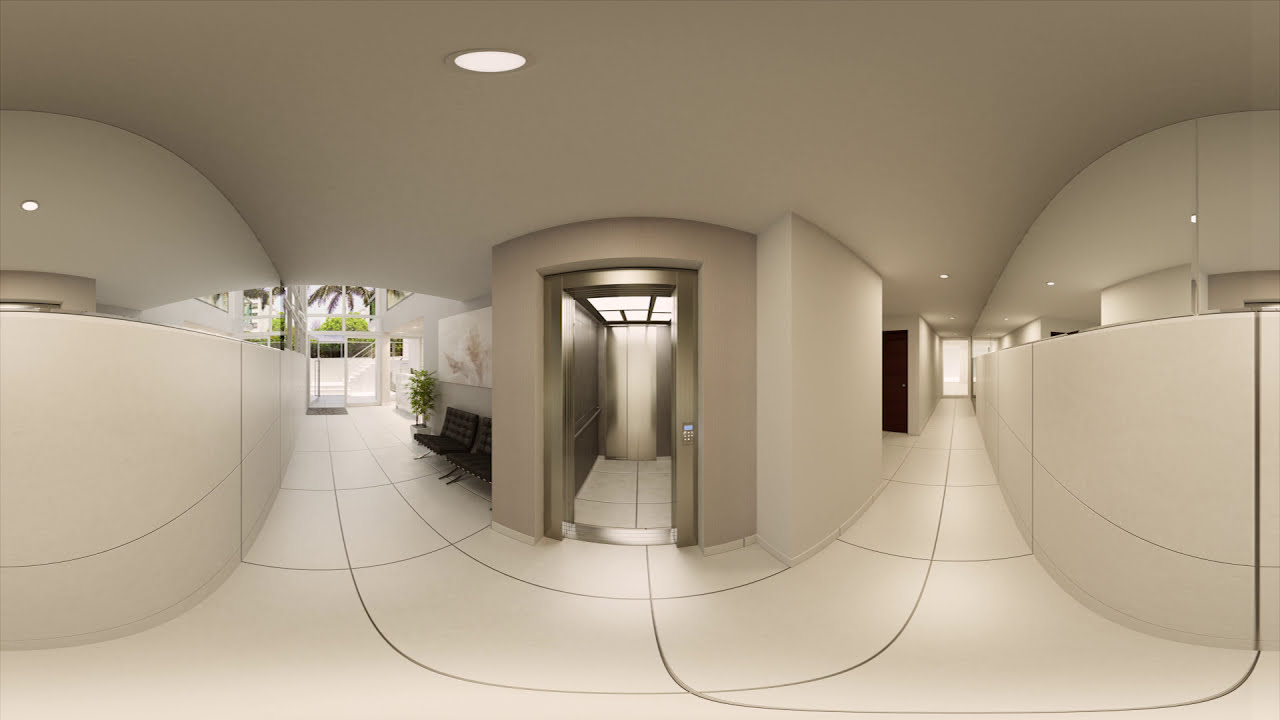This panoramic color photograph captures a broad view of a sleek, modern hotel or apartment building lobby. Predominantly featuring curved, white walls and a clean white floor that seamlessly flows through the space, the image is divided into three sections. At the center, an open elevator with a metallic, stained glass door frame stands as the focal point. The elevator’s interior mirrors the white flooring, exuding a minimalist aesthetic. Curved walkways extend from the elevator into the background, flanked by clear, window-like doors that lead outside, where tall potted plants are visible. Recessed lighting in the ceiling subtly illuminates the left side of the frame. The left segment of the panoramic view shows a cream-colored, rounded counter under overhead lighting and cushioned benches for seating. The right section offers another perspective on this counter. The entire space feels meticulously designed for both form and function, with elements of photographic representationalism and realism highlighted by fisheye and panoramic filters. No people or pets are present in this serene, meticulously clean environment.